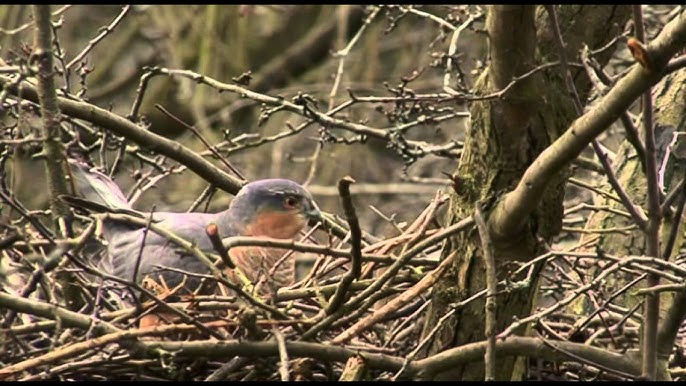The photograph captures a detailed, realistic image of a bird nestled within a round, bowl-shaped nest made of intertwined beige and brown twigs. The bird, positioned on the left side of the image and in profile facing right, exhibits a striking plumage. Its back and the top of its head are a bluish-gray, while its long, pointed black beak and dark crowned head accentuate a contrast with its orange throat and chest decorated with subtle white stripes. The bird's tail feathers are a mix of gray and white, pointing towards the top left. The nest rests on a thin-trunked tree with multiple bare branches extending outward, adorned with patches of light green moss. In the background, more leafless trees and branches create a rustic, forested backdrop, enhancing the natural setting of the scene. The photograph is rectangular in shape and oriented in landscape, embodying a photographic representationalism style.